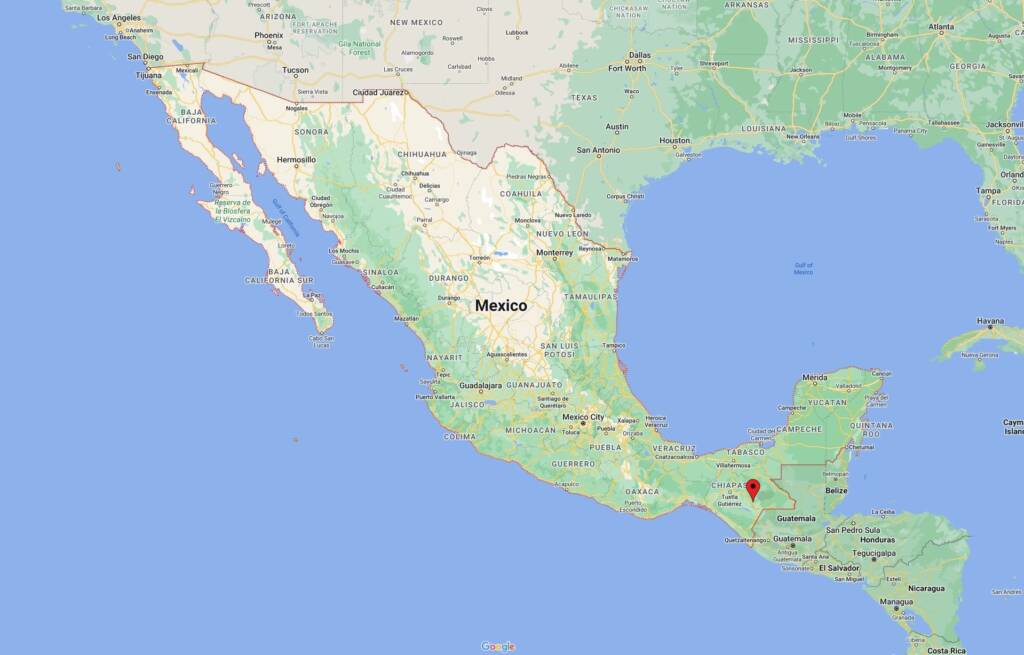This detailed map showcases the southern part of the United States, extending into parts of Central America, with a focus on both topography and key urban areas. The water bodies, including the Pacific Ocean and the Gulf of Mexico, are vividly depicted in blue. Land regions feature colors indicating topographical variations, with green and white dominating the landscape.

In the United States, the map highlights the lower halves of California, Arizona, New Mexico, Texas, Mississippi, Louisiana, Alabama, Georgia, and Florida. Portions of Arkansas are also visible. State boundaries are delineated by black lines, while major highways and roadways are marked with yellow lines. Prominent cities are clearly indicated, including:
- In California: Los Angeles and San Diego
- In Arizona: Phoenix and Tucson
- In New Mexico: Albuquerque (it's slightly obscured)
- In Texas: Austin, San Antonio, Houston, Dallas, Fort Worth, and Lubbock
- In Mississippi: Jackson
- In Louisiana: Shreveport and New Orleans
- In Alabama: Birmingham and Montgomery
- In Georgia: Atlanta, Augusta, and Savannah
- In Florida: Jacksonville, Tallahassee, Orlando, and Tampa

Additionally, a portion of Cuba is visible, featuring Havana, located just south of Florida.

The map also covers parts of Mexico and Central America. Significant Mexican cities marked include Guadalajara, Mexico City, Chihuahua, Sonora, Puebla, and Veracruz. A notable red dot marks Chiapas, situated just above Guatemala in the southern region of Mexico. Central American countries such as Belize, Honduras, Nicaragua, El Salvador, and Costa Rica are also represented.

Overall, this map offers a comprehensive view of the southern United States and neighboring regions, emphasizing geographic details and urban centers.